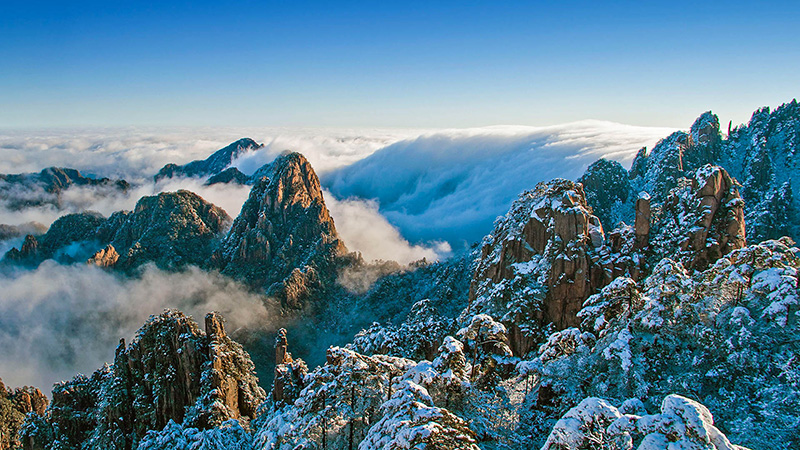This is an aerial photograph capturing the awe-inspiring spectacle of a towering mountain range. The rocky, craggy peaks are cloaked in snow, giving a striking contrast of white against the brown and granite hues of the stone. The scene is set at an extremely high elevation, evident from the myriad of clouds floating amongst and just below the peaks, creating a mesmerizing, almost ethereal view. The mountains shoot up through a dense blanket of clouds that rolls in like solid fog, adding a dynamic, water-like appearance to the landscape. The sky above is a gradient of colors, transitioning from a pale blue near the cloud layer to a deep, dark blue at the top, completely clear and devoid of clouds. The horizon is a vast expanse of blue, with hints of light gray where the sky meets the distant clouds. There are no signs of trees or vegetation, reinforcing the sheer altitude of the scene. The entire vista extends from the foreground, where snow-covered rock formations dominate the view, to the distant background, where the misty clouds continue to cascade over the grand peaks, creating an utterly captivating and otherworldly panorama.